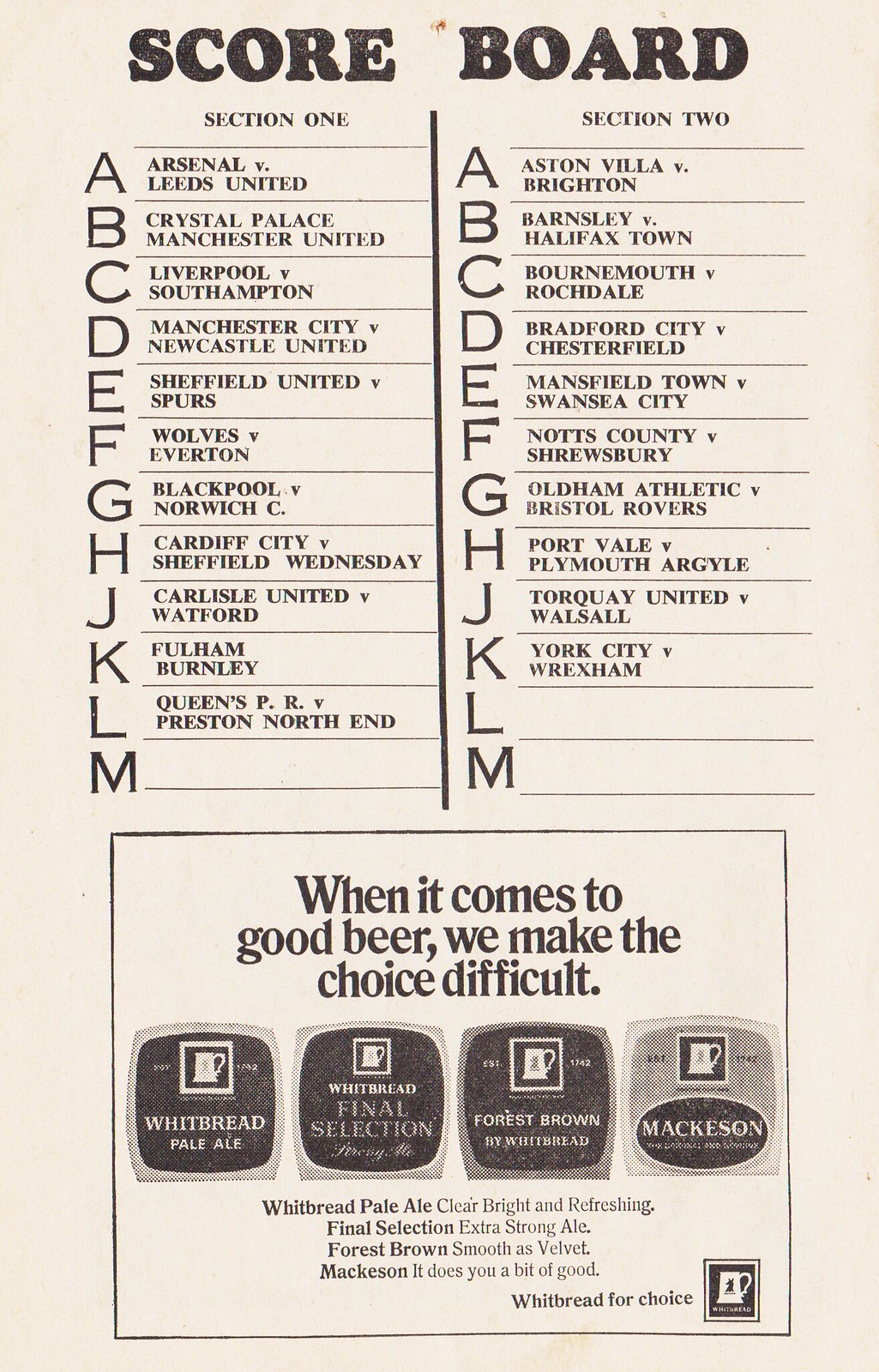The image depicts an off-white piece of paper with the heading "SCOREBOARD" in large, bold letters at the top. The layout features two separate sections labeled "Section 1" and "Section 2," each with columns marked A through M. Each letter corresponds to a different match-up. For example, in Section 1, A is Arsenal versus Leeds United, B is Crystal Palace versus Manchester United, C is Liverpool versus Southampton, and D is Manchester City versus Newcastle United. In Section 2, A is Aston Villa versus Brighton, B is Barnsley versus Halifax Town, and C is Bournemouth versus Rochdale, with teams continuing to be listed alphabetically. At the bottom of the page, there is an advertisement for a beer company that reads, "When it comes to good beer, we make the choice difficult," showcasing five different beer offerings. The overall design of the page suggests it may date back to the 1970s or early 1980s.